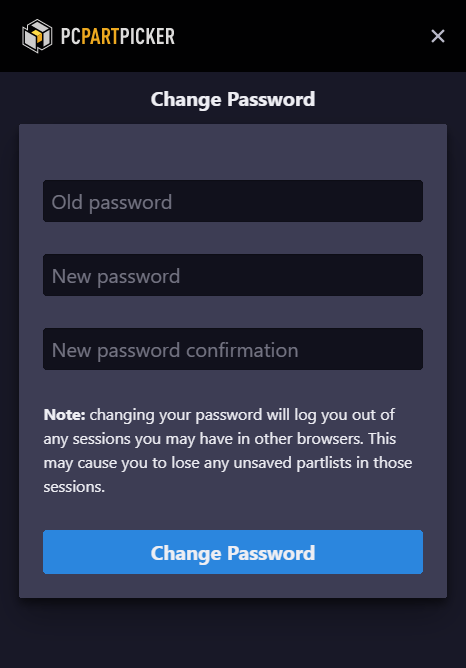The image depicts a user interface for PC Part Picker on a background that is entirely black. Prominently centered is a gray rectangular box containing relevant information. In the top left-hand corner of this box, "PC Part Picker" is written with "PC" and "Picker" rendered in white, while "Part" stands out in orange; the words are fused together.

To the left-hand side of the box, there is a white icon resembling an open box with an orange strip through the middle. In the upper right-hand corner, a white "X" symbol is visible, indicating a button to close the window. Below the title, the interface is clearly arranged for changing a password.

The form includes distinct fields labeled "Old Password," "New Password," and "New Password Confirmation," allowing users to input the appropriate information.

Above these fields, there is a note in white text, prefaced by two semicolons: "Note: Changing your password will log you out of any sessions you may have in other browsers. This may cause you to lose any unsaved part lists in those sessions."

The interface is topped off with a blue bar at the bottom, featuring the words "Change Password" in white, indicating the action button for the form.